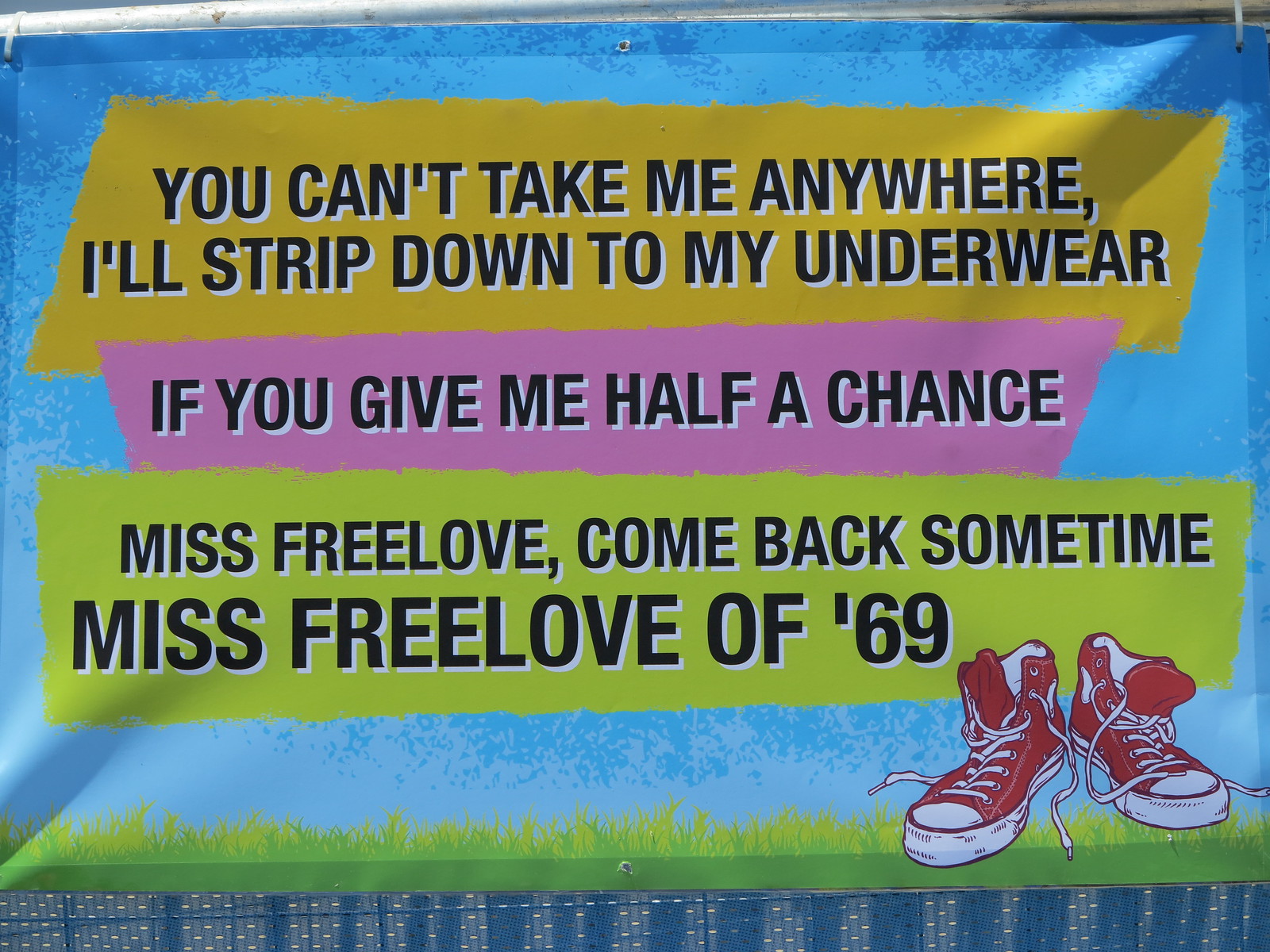The image depicts a vibrant and colorful banner with a light blue background. At the very top, in a yellow text box with bold black letters, it reads, "You can't take me anywhere. I'll strip down to my underwear." Below, in a pink text box with large black bold letters, it says, "If you give me half a chance." The bottom portion features a lime green text box with the inscription, "Miss Free Love, come back sometime. Miss Free Love of 69." The banner is accentuated with a base of cartoonish green grass along the bottom edge. In the bottom right corner, there is an illustration of a pair of red sneakers with white laces and white toe caps, appearing slightly worn and disheveled. The banner is likely displayed on a pole, allowing it to hang down prominently.